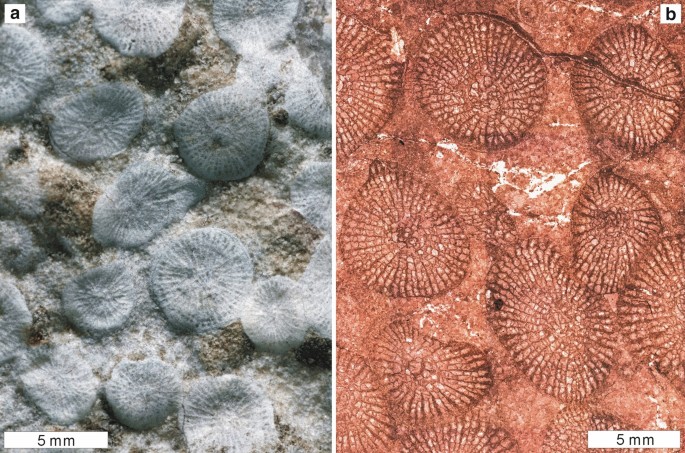The image is presented as a split screen, with two separate sections marked as A and B at the top left and top right corners, respectively. Both images feature a "5MM" scale marker in the bottom corners, indicating the measurement reference. 

On the left (Image A), a collection of circular objects is visible, predominantly in a bluish-gray hue with light brown interspersed areas. The circles, appearing delicate and almost bubble-like, rest on a thick, fuzzy surface. This side suggests an underwater or microscopic view, possibly depicting small sea organisms or bacterial colonies with a nuanced texture.

On the right (Image B), the scene transforms, showing the same circular objects, but now bathed in an orange-red tone. The image appears slightly zoomed in, emphasizing the circle’s texture that radiates from the center outward. There are eight circles clearly positioned at the bottom and three near the top, with some partially cut off, maintaining the detailed, delicate structure seen in the left image.

These comparisons suggest that the two images might be of the same materials under different staining processes or imaging techniques, demonstrating the variation in color and texture between the two views.